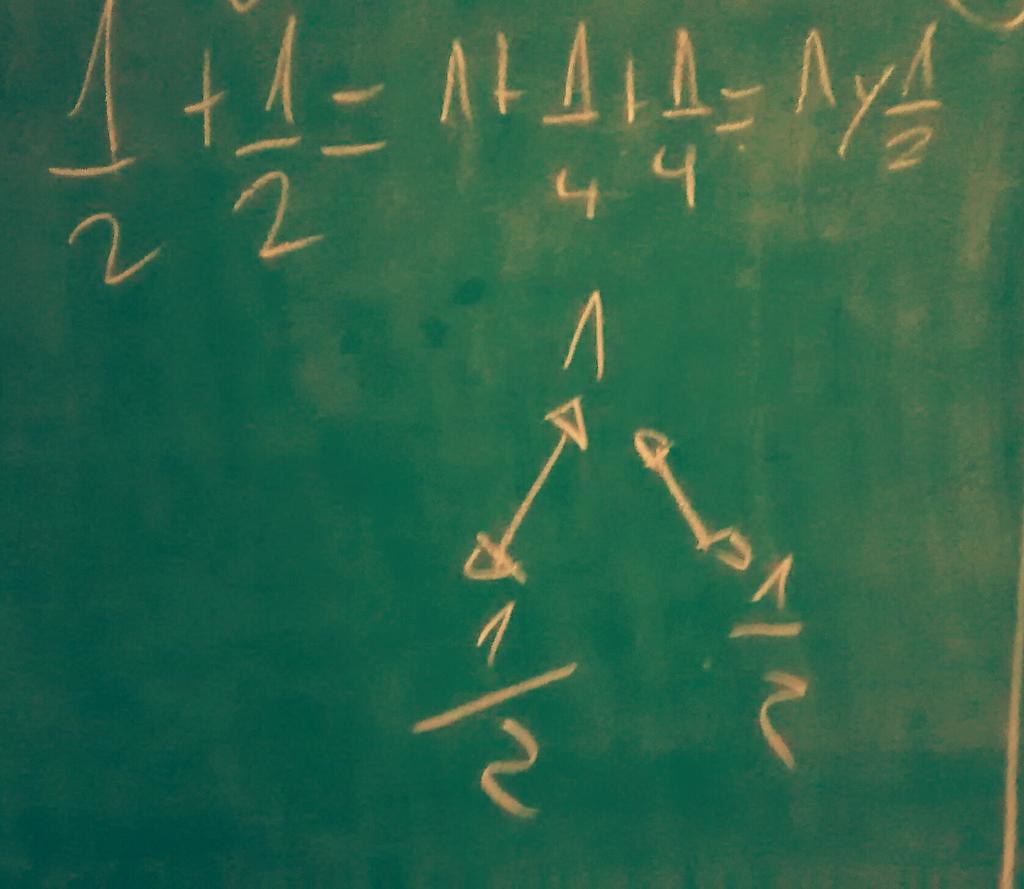The image depicts a green chalkboard marred by a variety of eraser marks and stains, giving it an uneven appearance with areas of darker green. Scrawled upon the board in yellow chalk is a complex formula that incorporates a recurring pointed symbol, resembling half of a triangle without a base. 

Starting from the top left, the sequence begins with this symbol over 2 added to the same symbol over 2, which collectively equals the symbol on its own. Below, the symbol reappears over 4, followed by another addition of the symbol over 4, summing up to the symbol once again. Further down, a combination of the symbol and another symbol appears over 2.

At the very bottom of the chalkboard, the same pointed symbol over 2 is displayed on either side of the board. Between these fractions, two thick chalk arrows, with open-ended points, bidirectionally connect the lower fraction to the upper fractions of the formula.

Notably, the upper right corner of the chalkboard shows signs of frequent erasures, indicating that parts of the formula in that area had been written, wiped out, and rewritten multiple times.